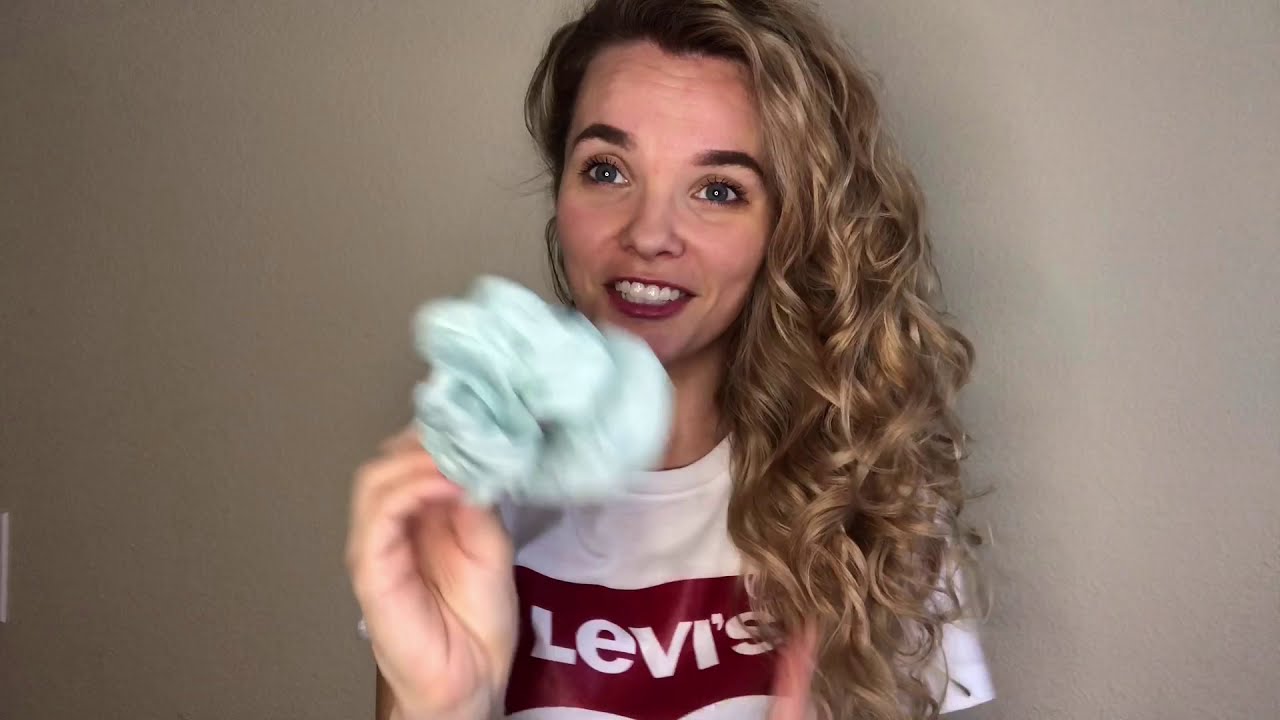In the center of the image stands a woman with long, wavy blonde hair that falls past her shoulders, characterized by large curls. She is slightly smiling, revealing her white teeth, and has bright blue eyes and thick dark brown eyebrows. Her lips are adorned with bright red lipstick. She is wearing a white short-sleeved t-shirt that prominently features the Levi's logo in bold red and white capitalized letters. In her right hand, she holds a crumpled light green fabric, possibly a mint green cloth or a light blue fluffy hair tie, and there might be a ring on her hand. The background behind her appears to be a solid color, likely tan or gray, giving the impression of a grave wall or a room. The image has a slight blurriness to it, adding a soft focus to the overall scene.